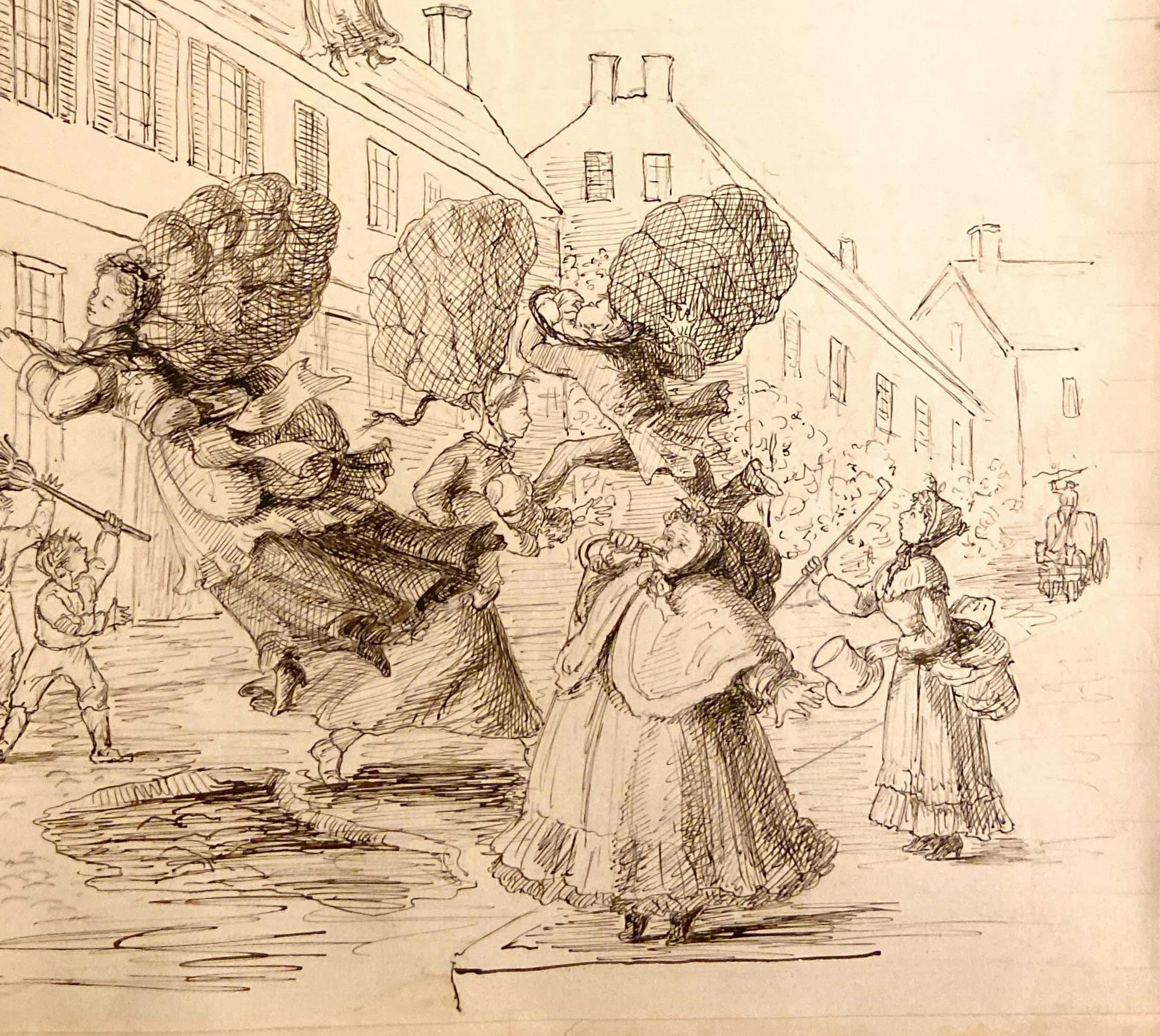This intricately detailed pencil drawing resembles an old political cartoon, likely from over a century ago, possibly from the 1800s. The scene depicts a bustling street filled with distinguished figures dressed in period attire. Elegantly dressed women, adorned in voluminous petticoats and bonnets, promenade alongside men sporting top hats.

Central to the image are three women who stand out from the crowd, each gripping a balloon in one hand and a large net in the other. These balloons seem to defy gravity, lifting the women slightly off the ground and creating a whimsical, almost surreal scene. Bystanders are depicted with startled expressions, their attention riveted on the floating women.

Several onlookers, equipped with canes, are actively attempting to reel the women back down, their actions suggesting a mix of concern and astonishment. The drawing captures a moment of unexpected levity and curiosity, providing a glimpse into the imaginative social commentary characteristic of period political cartoons.